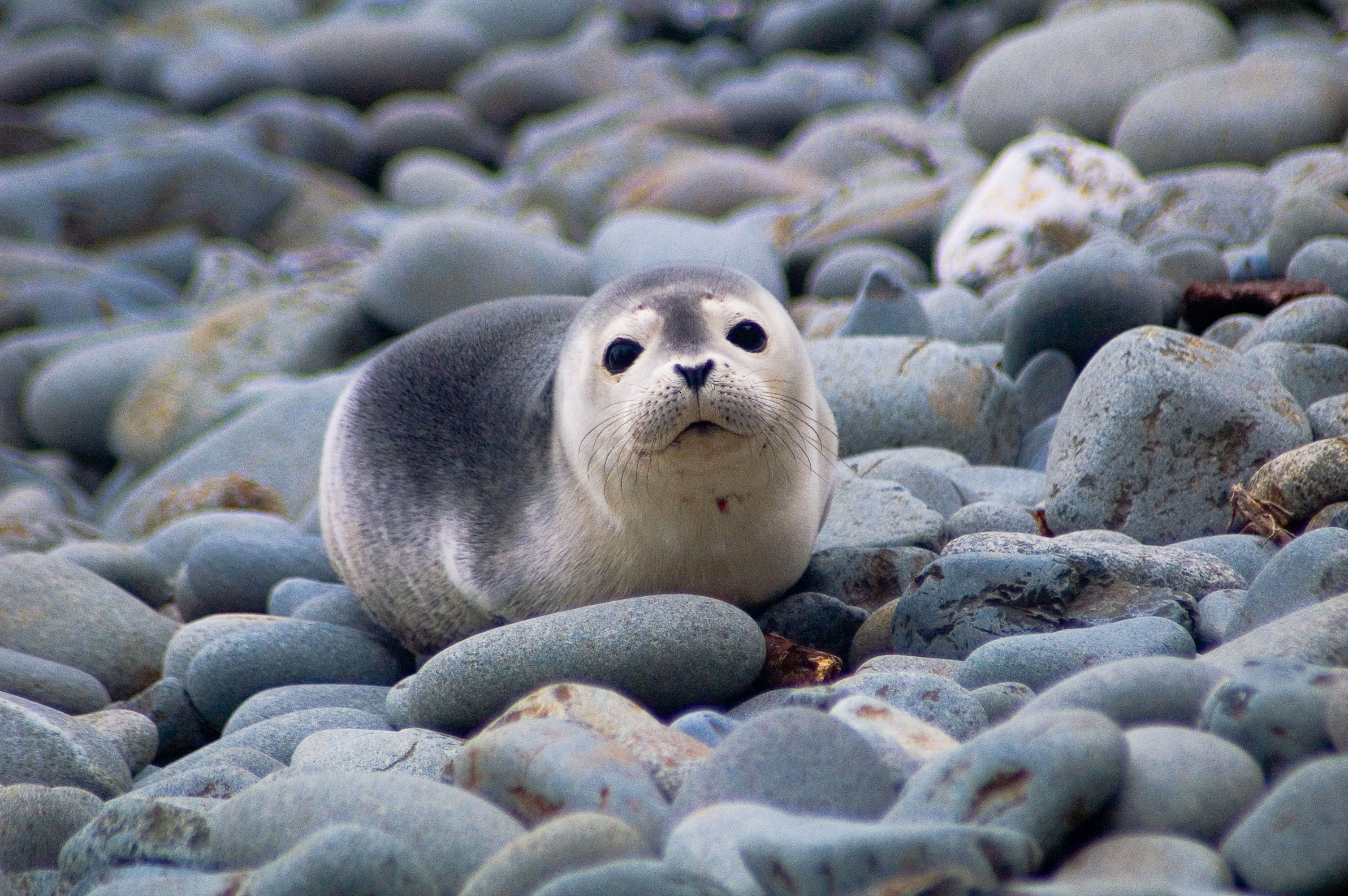In this detailed photo, a baby seal rests amidst a rocky shoreline. The environment is characterized by large gray stones, with varying textures and intermittent specks of green. Some rocks exhibit golden hues or brown crevices, adding depth to the scene. The baby seal, positioned slightly to the left of center, has a captivating appearance. Its fur transitions from a dark gray on its back and the top of its head to a lighter gray and then white towards its belly. The dark gray extends between its large, expressive black eyes, down its muzzle, to its black nose shaped like an upside-down pyramid. The seal's legs or flippers are tucked beneath its body, and it has a multitude of small black whiskers adorning its face, with visible whisker holes. The seal gazes directly at the camera, seemingly focusing on the photographer. The background rocks become increasingly blurry, emphasizing the seal pup in the image's foreground.